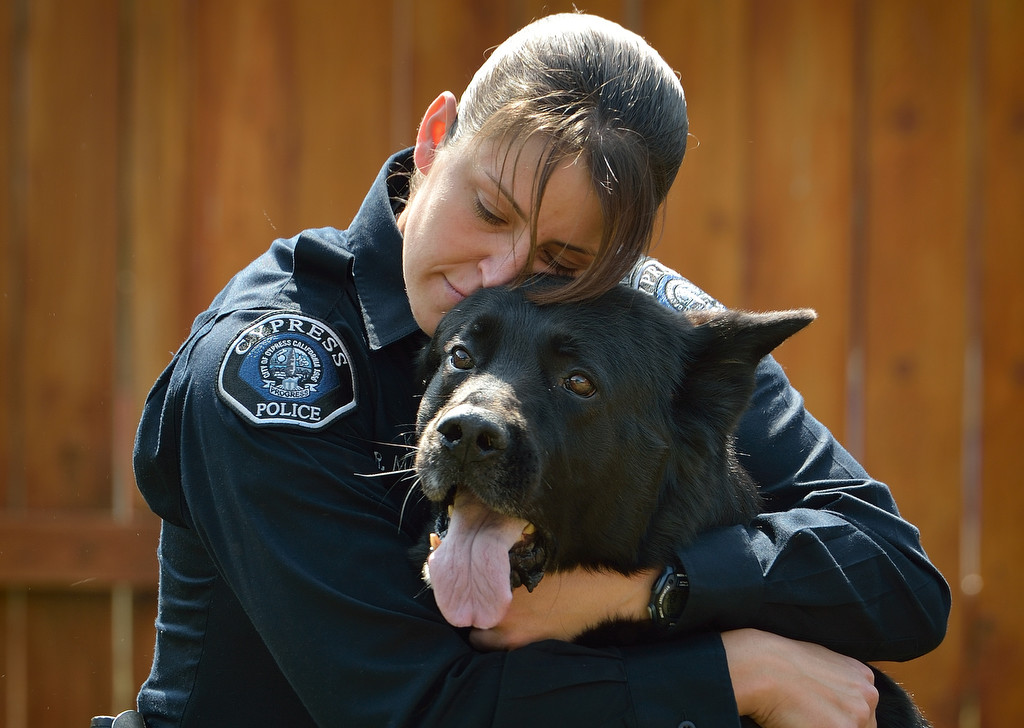In the image, a young policewoman, possibly in her late twenties to early thirties, is seen embracing a large black dog reminiscent of a Labrador, often used as a drug-sniffing dog. The policewoman is wearing a black uniform with a shoulder pad that displays the label "Cypress Police." She is crouched down, likely seated on the ground, with her head resting on the dog's body and her arms wrapped around it in a warm embrace. Her brown hair is tied back with a long fringe swept across her forehead, which does not obstruct her vision. The dog, with its pink tongue hanging out, is gazing attentively into the distance with its expressive brown eyes. Behind them, a wooden slatted fence forms the backdrop, slightly blurred, which emphasizes the clear and sharp focus on the tender moment shared between the policewoman and her canine companion. The woman appears emotionally attached to the dog, highlighting a bond of affection and trust. The woman is of Caucasian appearance, and her posture and facial expression convey a profound sense of camaraderie and care toward the diligent dog in her embrace.